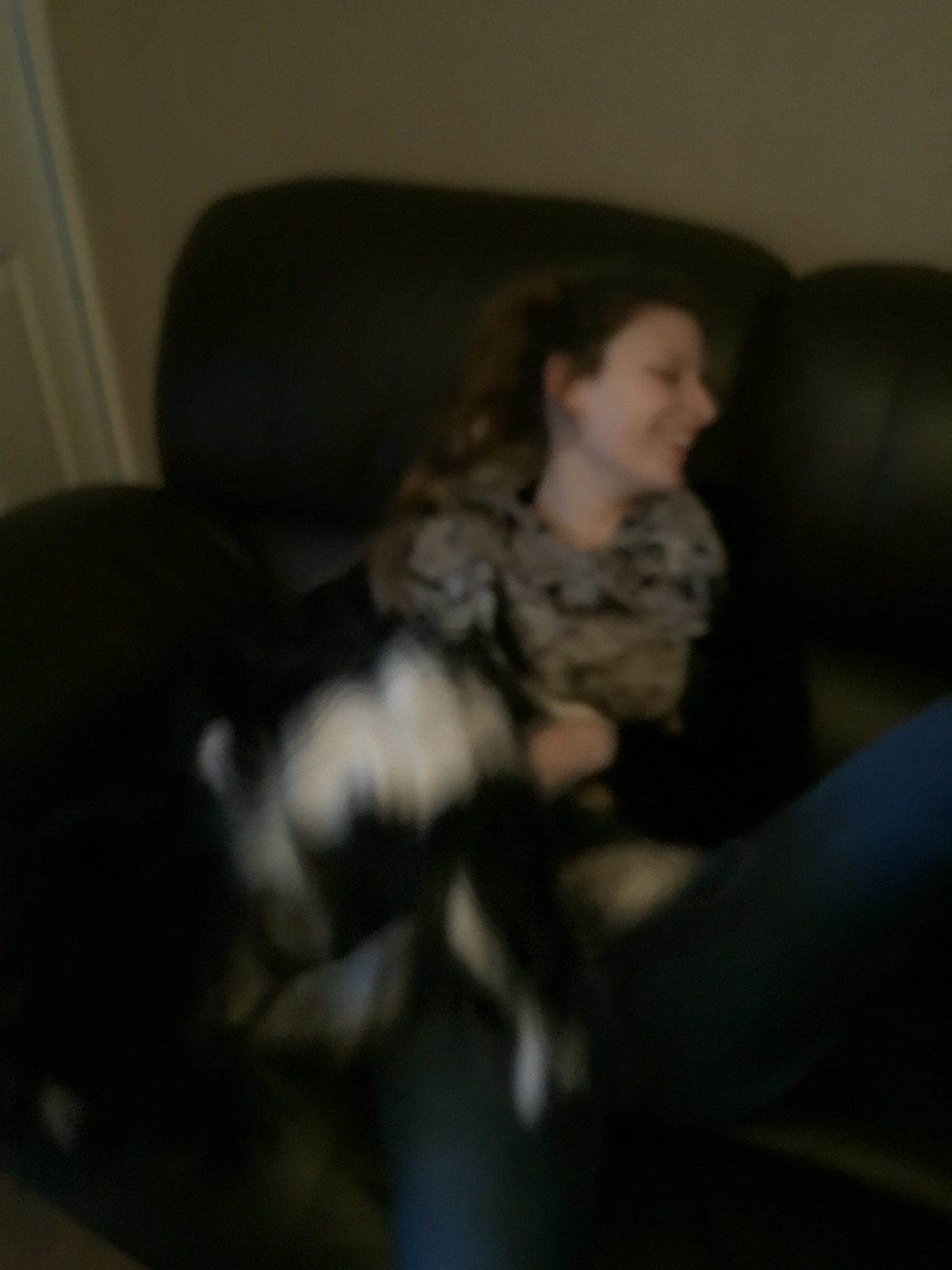This photograph, though of very low quality and heavily blurred, captures a dynamic moment. The image was likely taken while either the photographer or the subject were in motion, resulting in the significant blur. At the center of the frame, a woman with her hair pulled back into a ponytail can be seen. She is wearing what looks like a scarf around her neck and has her face turned in profile as she looks to her left, smiling and appearing content. In her lap, there is a black and white animal, possibly a dog, which seems to be wriggling, attempting to escape her grasp. The woman is seated on a couch, providing a relaxed backdrop to this otherwise fleeting moment.